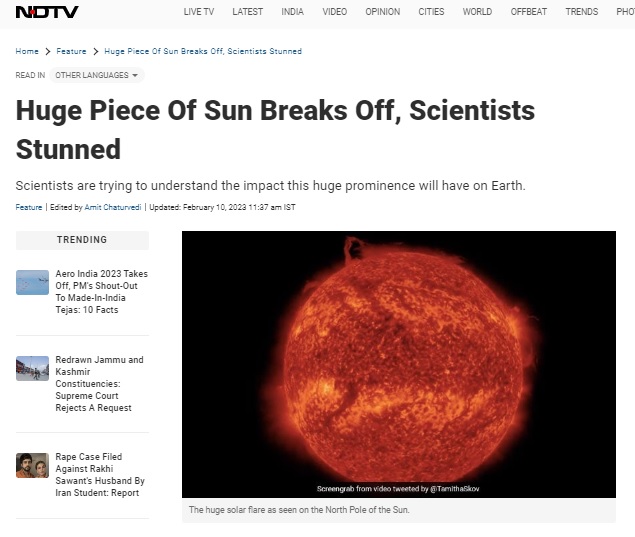The image features a screenshot of a news website with a gray background at the top. The headline area is marked by the NDTV logo in black, with a distinctive red circle placed between the 'N' and 'D'. Below the logo, there is a navigation bar with a blackish-purplish hue that lists several tabs, including "Live TV," "Latest," "India," "Video," "Opinion," "Cities," "World," "Offbeat," "Trends," and a partially obscured tab labeled "PHO," likely short for "Photos."

Further down, a featured article is prominently displayed with the headline "Huge Piece of Sun Breaks," followed by a subtitle reading "Scientists are trying to understand the impact this huge phenomenon will have on Earth." The article mentions that it is edited by someone named "Chaturvedi," with the text displayed in light blue. The publication details indicate that the article was updated on February 10th, 2023 at 11:37 a.m. IST.

On the left side of the page, there is a "Trending" section listing several articles: "Aerial India 2023 Takes Off," "PM Shout Out to Made in India Tejas," "Ten Facts," "Redrawing Jammu and Kashmir Constituency," "Supreme Court Rejects the Request," and "Rape Case Filed Against Rahi Sawai's Husband by an Iranian Student."

At the center of the image, there is a photograph depicting a large, brightly colored solar flare, with red and orange hues set against a black background. The caption below the image states: "The huge solar flare as seen on the north pole of the sun."

This detailed description encapsulates the various elements present in the image, providing a comprehensive overview of the visual content and text.